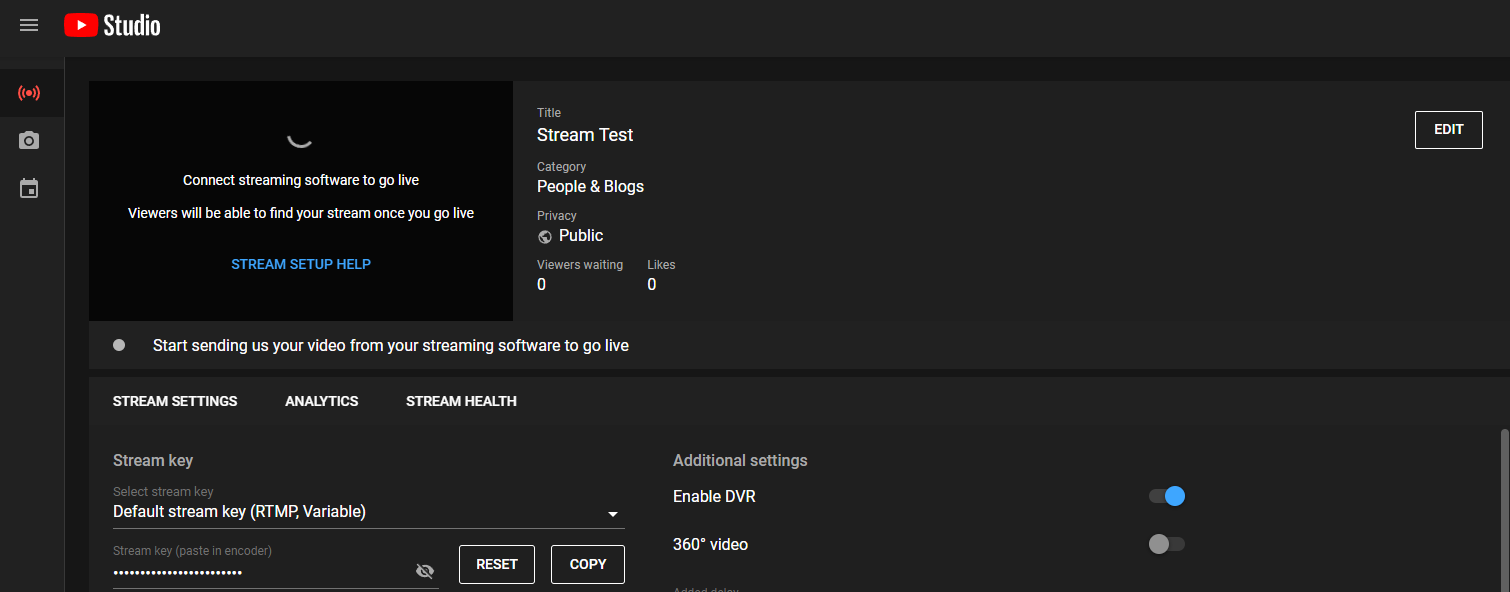The image shows the YouTube Studio interface, specifically the live streaming setup page. At the top-left corner, there is the YouTube logo—a red rectangle with a white play button inside—next to which it reads "Studio." The background of the interface is a dark slate gray, almost black. 

Beneath the top-left corner, there is a menu icon consisting of three horizontal lines, followed by several tabs: a dot with lines on either side, a photo icon, and a calendar icon. The tab with the red dot and lines seems to be currently selected.

The main section of the interface instructs users to "Connect streaming software to go live," explaining that viewers will be able to find the stream once it starts. A blue hyperlink labeled "Streaming setup help" is placed below this instruction, presented in white text on a black background.

To the right, there are additional details such as the stream category, indicated as "People & Blogs," and the privacy setting marked as "Public." There are also status indicators for "Viewers Waiting" and "Likes," both currently showing zero.

Just below, the interface prompts the user to start sending video from their streaming software in order to go live. 

Further down, there are options and information regarding stream settings, stream analytics, stream health, and the stream key. It mentions the "Default Stream Key" with the label "(RTMP, variable)." An area marked "Stream Key" shows a pasted key obscured by dots with an "I" that has a line through it, for security purposes. There are options to "Reset" or "Copy" the stream key.